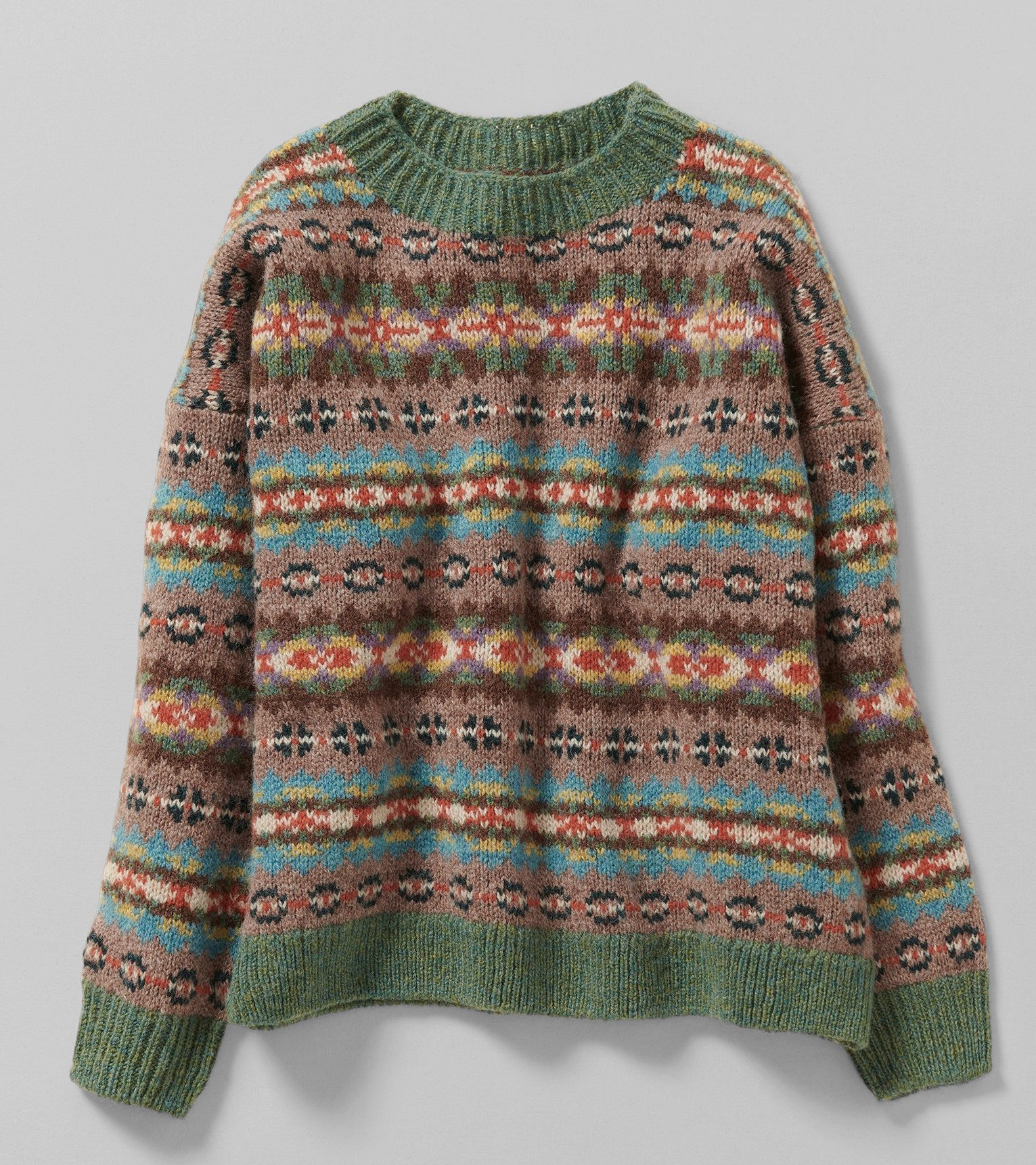This image depicts a handmade knitted sweater set against a light gray background. The sweater is predominantly tan with various intricate horizontal patterns in multiple colors such as beige, brown, blue, red, yellow, and black, giving it a vibrant and chaotic tapestry-like appearance. 

The neckline, wrist cuffs, and waist band are all ribbed with a distinct light green color, though the knit of the waistband appears tighter and less ribbed compared to the neckline and cuffs. Just below the collar, there is a light pink stripe decorated with green circles featuring red dots in the center. Further down, below the armpits, there is another horizontal stripe adorned with red circle patterns that resemble suns, with X's interspersed between them. In the middle section, a light blue-teal horizontal band accented with yellow dots adds another layer of detail to the sweater's eclectic design. 

This intricately knit piece, likely made from wool, stands out for its varied geometric patterns and bold use of colors, combining elements that seem almost floral yet remain distinctly abstract.